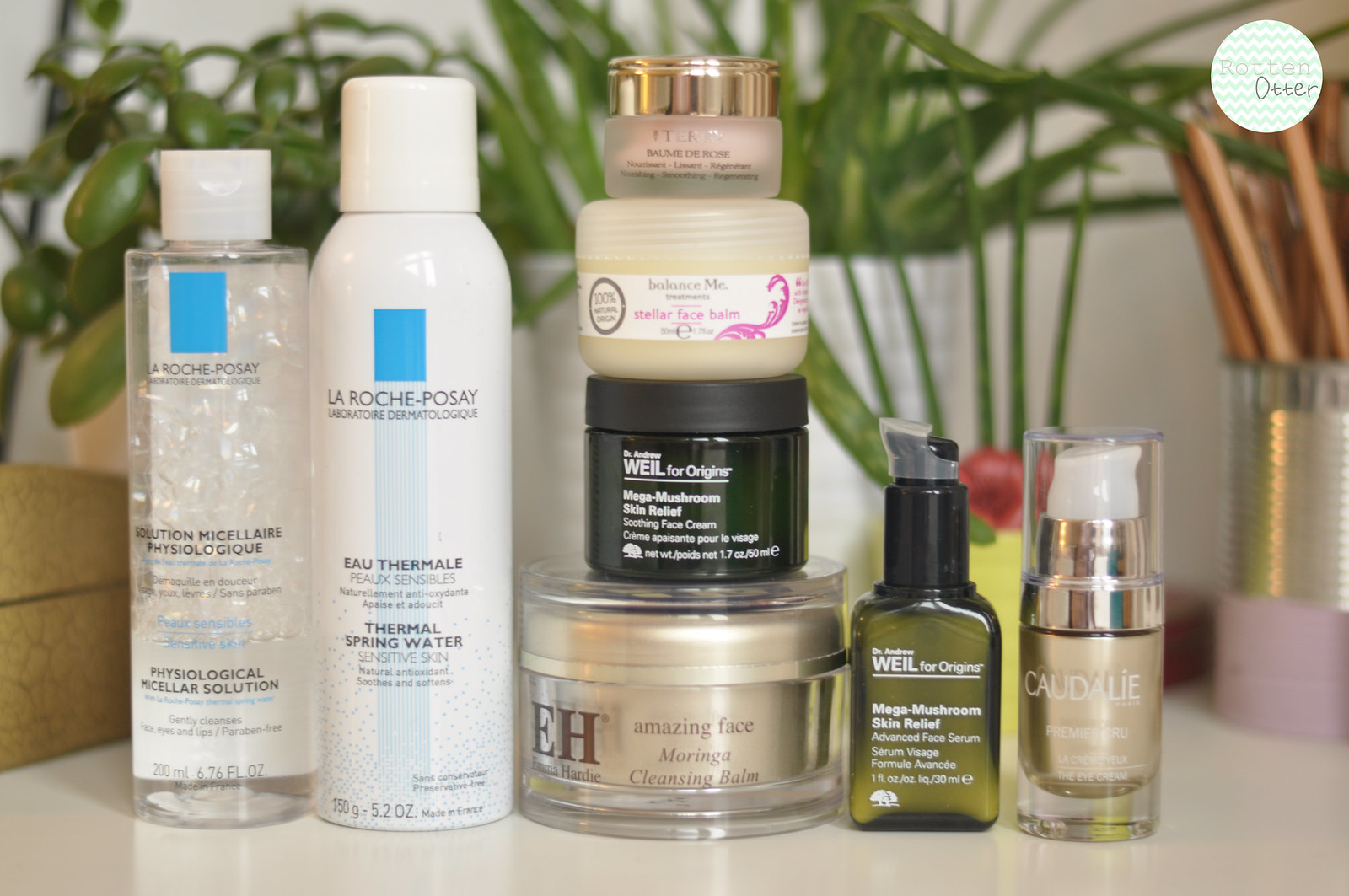The image showcases a selection of beauty products arranged on a pristine white countertop. The backdrop features a minimalistic white wall, complemented by the presence of a lively green plant in a sleek white pot, infusing a touch of nature into the scene. 

On the left-hand side, there is a brownish box, setting a warm contrast to the white surroundings. The centerpiece of the display is a collection of La Roche-Posay products. Among them is a clear bottle of Micellar Solution, showcasing its transparency. Adjacent to it is a white can of Thermal Spring Water, characterized by its opaque exterior.

A stack of four products draws attention at the center. At the bottom lies a cleansing balm, topped by a jar of Mega-Mushroom Skin Relief Soothing Face Cream. Above it sits a Stella Face Balm, and at the very top is a small, indiscernible product adding a final touch to the neatly arranged stack.

To the right of the stack, there is a green bottle of Mega-Mushroom Skin Relief Men's Face Serum. Finally, a product housed in a gray bottle with a white pump top completes the array, its modern design contrasting subtly with the other items.

The harmonious arrangement and varied textures of the products, along with the natural element of the green plant, create a visually appealing and serene composition.